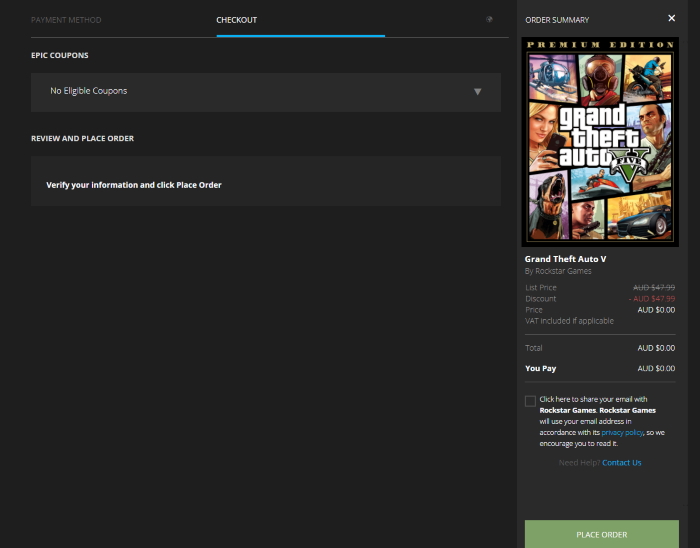Here's a detailed and cleaned-up version of the caption for the image:

---

The screenshot captures a checkout screen from a website or app, featuring a dark gray to black background. At the top left corner, there are two tabs labeled "Payment Method" and "Checkout," with the "Checkout" tab highlighted by a blue underline to indicate it is the selected option. Adjacent to these tabs on the right side, there is a small globe icon.

Beneath the tabs, a section titled "Epic Coupons" is visible, containing a dropdown menu with a downward-facing triangle that reads "No eligible coupons." Following this section, there's a prompt stating, "Review and place order. Verify your information and click place order."

On the right-hand side, a vertical bar takes up approximately one-quarter of the page's width. This segment is labeled "Order Summary" and provides the details of the purchase. The item listed is "Grand Theft Auto V," specifically the Premium Edition by Rockstar Games. The summary includes the original list price as AUD $47.99, a discount of AUD $47.99, and the final price of AUD $0, VAT included where applicable. Consequently, the total amounts to AUD $0, indicating that no payment is required.

Also within the order summary, there is a checkbox option allowing users to share their email address with Rockstar Games, alongside a note encouraging users to read the privacy policy. It also offers a reminder to contact customer support if help is needed.

At the bottom of the screen is a prominent green button labeled "Place Order," guiding users to finalize their purchase.

---